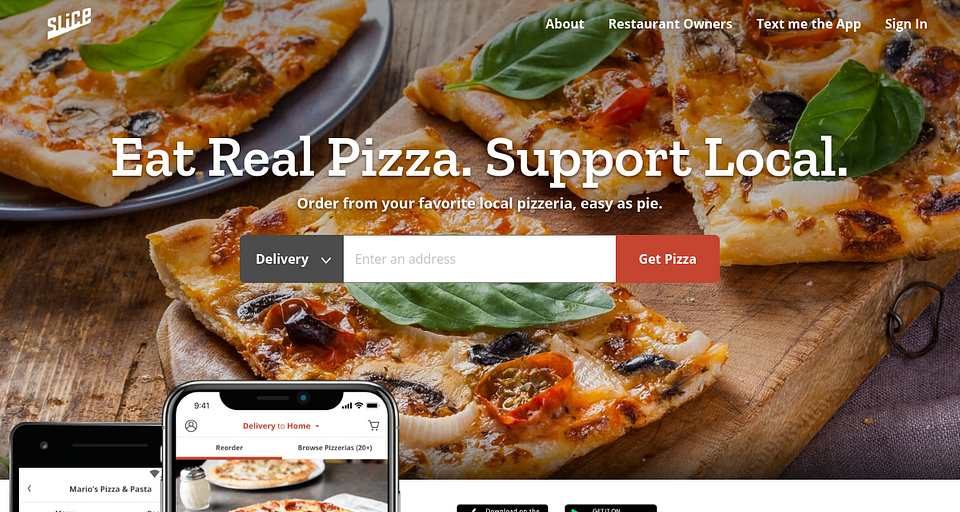This is a detailed screenshot of a cleverly designed advertisement masquerading as a website. The background of the page features a rustic aesthetic, with wooden planks topped with slices of pizza, creating a homey yet unappetizing atmosphere. The pizza appears unappealing with its gummy and dry texture, adorned with cheese, green peppers, white onions, and a single uncooked basil leaf per piece. Notably, the pizza slices are cut into squares rather than the traditional wedges.

In the upper-left corner, there is a blue ceramic plate holding a slice of this same pizza, adding to the overall pattern of food presentation. The name of the website, "Slice," is prominently displayed in the upper left, underlined in white for emphasis. 

The upper right corner of the screen features navigation options in white font, including "About," "Restaurant Owners," "Text Me the App," and "Sign In." 

Dominating the center of the image is a bold and inviting slogan: "Eat real pizza. Support local. Order from your favorite local pizzeria. Easy as pie." 

Directly below this call to action is a prompt for the user to "Enter an address" to get pizza, accompanied by a clickable red button, encouraging immediate interaction with the ad.